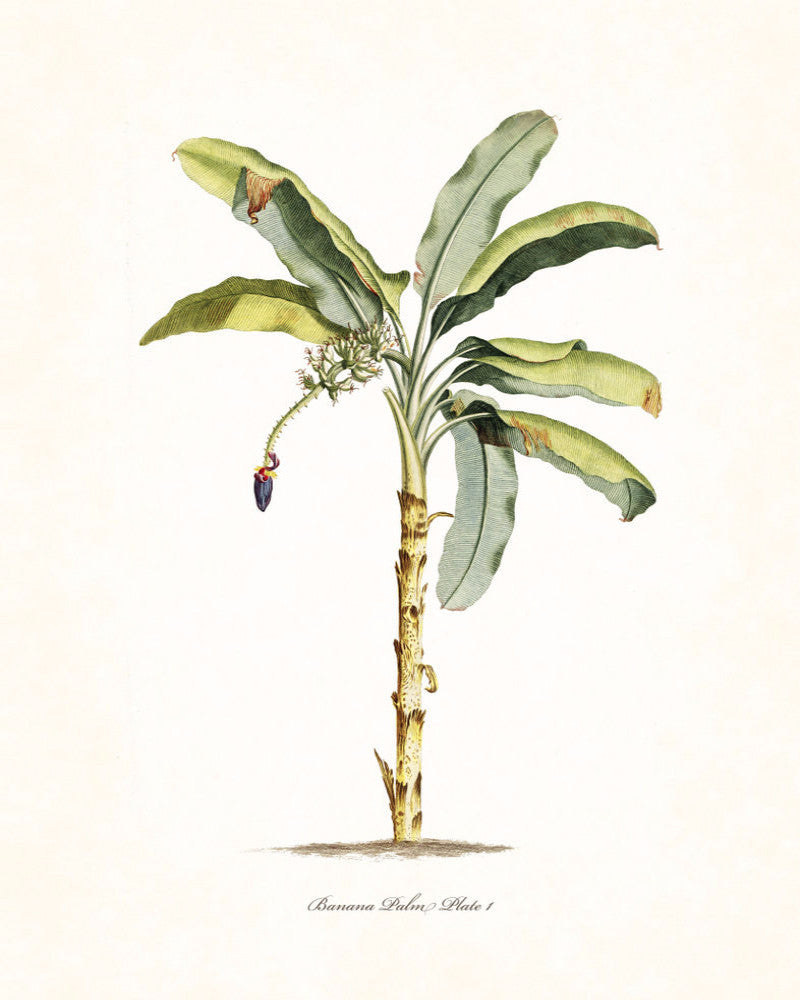The image is a detailed drawing of a banana palm, centrally located with a rectangular shape twice as tall as it is wide. The background is a light tannish-white color, resembling aged paper. The plant features a robust yellowish trunk with sections where the bark spreads outward, interspersed with dark brown patches. At the base, a small patch of dirt signifies its grounding. Crowning the trunk are multiple large, oblong, bean-shaped green leaves, with a few in a state of browning and withering. A prominent single stem emerges from the center, showcasing multiple white flowers. Additionally, a smaller branch from the top right bears a blue bud, distinct from the green foliage. Below the plant drawing, in elegant cursive text, it reads "Banana Palm Plate One."